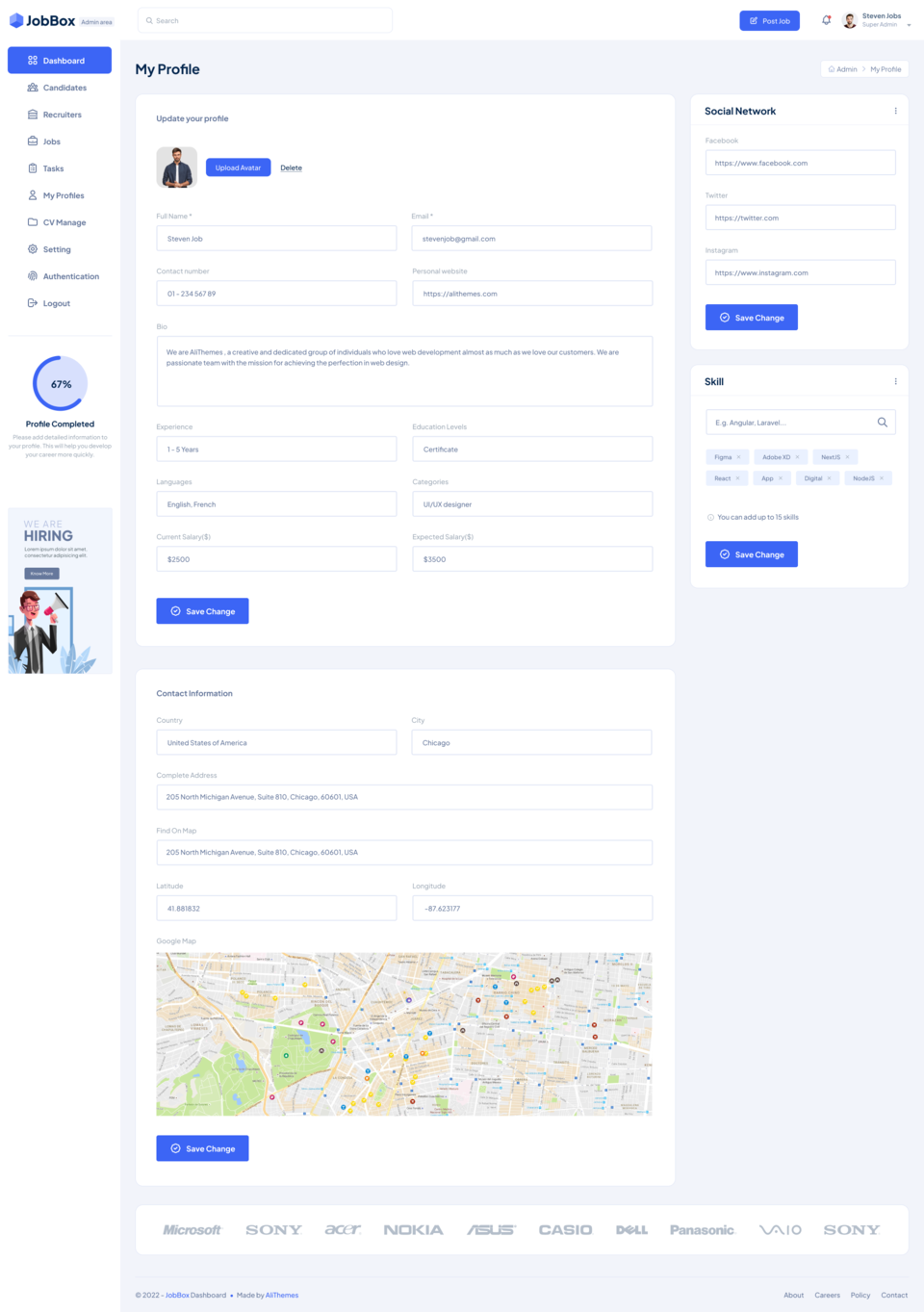The image displays the homepage of a job-search website named "JobBox." 

At the top of the page, there is a white background with the website's logo on the left: a blue cube with the text "JobBox" written as a single word. To the right of the logo, a search bar is prominently placed. Further to the right, there is a button labeled "Post Job," followed by a profile section that displays an image of Steven Jobs, accompanied by his name. Next to the profile section, an icon resembling a bell is visible with a red notification circle.

On the left-hand side, a vertical navigation menu is presented with several options. The "Dashboard" tab is highlighted in a blue-purple color, indicating it is the current selection. The menu also lists the following options: Candidates, Recruiters, Jobs, Tasks, My Profiles, TV Manage, Setting, Authentication, and Logout. A progress bar beneath the menu indicates that the user's profile is 67% complete.

In the main content area, a header reads "We Are Hiring." Below it, the section titled "My Profile" appears in bold black text. This section includes various editable fields for updating the user's information: Update Your Profile, Upload Avatar, Delete Full Name, Contact Telephone Number, Bio, Experience, Languages, Current Salary, Save Changes, Education Level, Categories, and Expected Salary.

Further down, another section labeled "Contact Information" asks for details such as Country, Complete Address, Find and Map, Latitude, Longitude, and City. At the very bottom of the page, an interactive map is displayed, with a "Save Changes" button situated beneath it.